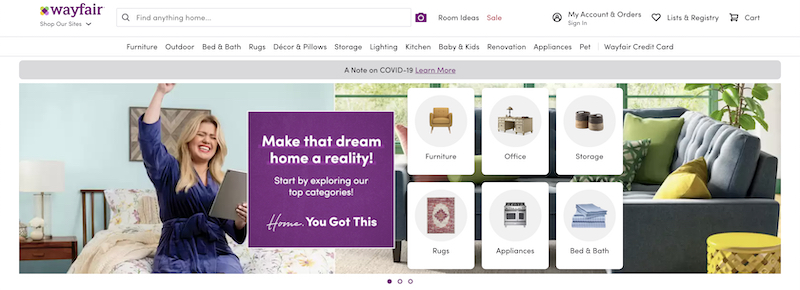The image is a screen capture of the Wayfair homepage. In the top left corner, the Wayfair logo is prominently displayed in purple. A search bar beside it invites users to 'find anything home,' adorned with a small magnifying glass icon. To the right of the search bar, options for navigating the site include a purple camera icon labeled 'Room Ideas,' a red 'Sale' notification, and links titled 'My Account,' 'Orders,' and 'Sign In.' Further to the right, tabs for 'List & Registry' and a shopping cart icon with the word 'Cart' are visible.

Directly beneath the primary navigation bar, black text categorizes the site’s offerings: 'Furniture,' 'Outdoor,' 'Bed & Bath,' 'Rugs,' 'Décor & Pillows,' 'Storage,' 'Lighting,' 'Kitchen,' 'Baby & Kids,' 'Renovation,' 'Appliance,' 'Pet,' and 'Wayfair Credit Card.'

Below these categories, a small gray horizontal rectangle provides a link to a note on COVID-19, marked by the text 'Learn More' in purple.

The main section of the screen features an image of a woman sitting on her bed, her arm raised in excitement. She has blonde hair and wears a blue robe. The woman is holding a tablet, sitting in a room with blue walls and a sofa to the right. The sofa is gray with various colored pillows, situated near a window. An overlaying purple square on the right side of the image reads 'Make that dream home a reality,' promoting Wayfair's offerings.